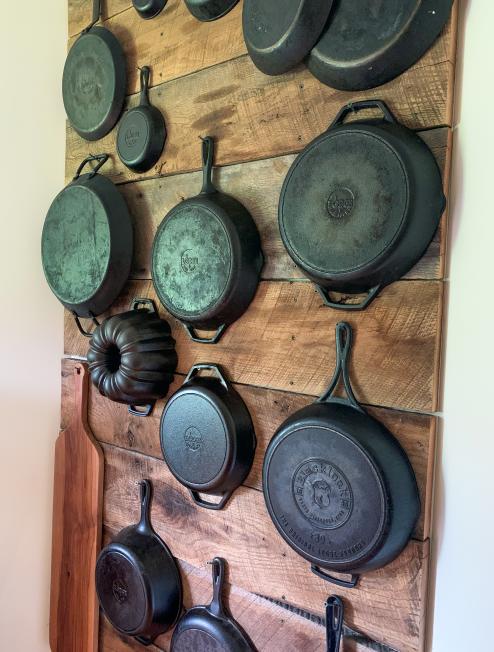The image depicts a light brown, horizontal-slatted, wooden display rack mounted on a white or pink kitchen wall. This wooden rack, possibly made of finished oak, is designed to hang various cast iron cooking materials, including different-sized skillets, pans, and a metal Bundt pan. Each item is hung on its own individual nail, with the cooking sides facing the wall, revealing the manufacturer's marks on the back. Additionally, a large wooden cutting board is hung vertically on the same backing. The skillets feature varying handle styles, with some having a single long handle and others having two side handles. The display showcases both new and used pieces, making for an organized yet varied kitchen setup.